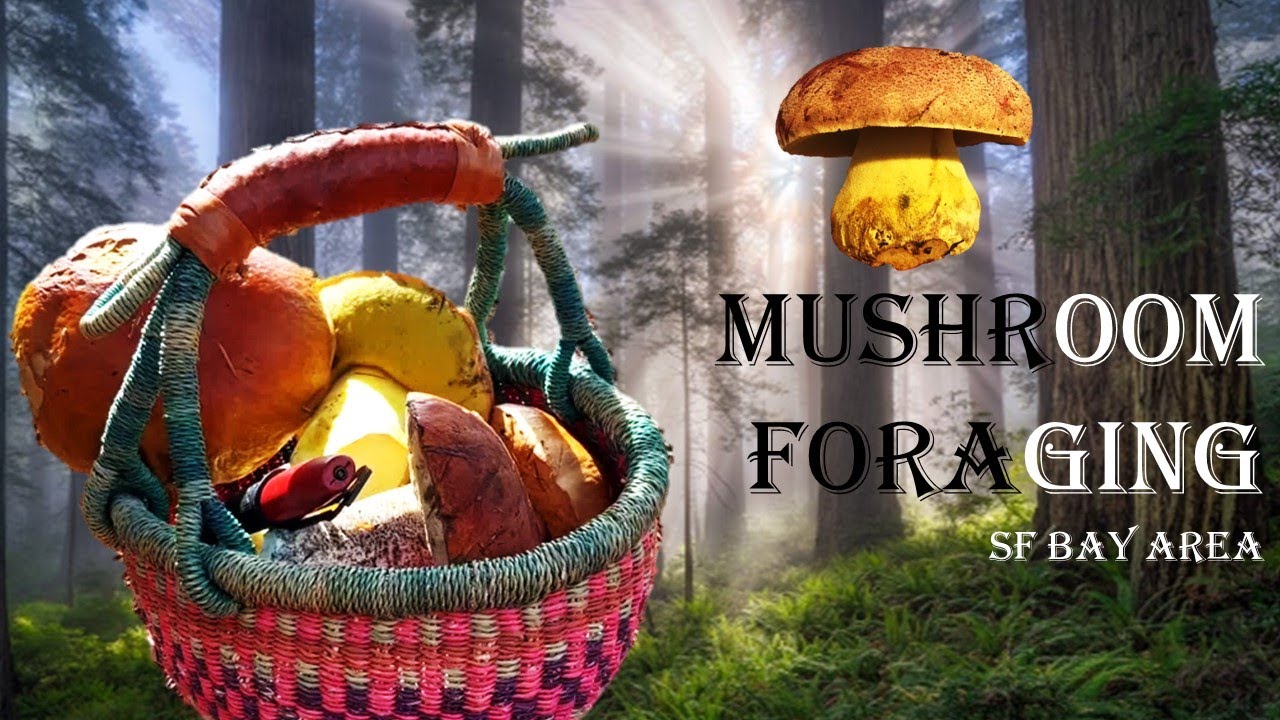The digital image appears to be crafted for an article or advertisement promoting mushroom foraging in the SF Bay Area. The background showcases a lush, foggy forest, likely from the Pacific Northwest, featuring majestic redwood trees with sun rays piercing through, mosses, grasses, and an overall prehistoric ambiance. Central to the image is a wicker basket with shades of red, pink, and bluish-gray on the rim. This basket is brimming with a diverse collection of mushrooms in various hues—yellow, orange, red, and brown. Prominently placed in the bottom right corner of the image is the text "Mushroom Foraging, SF Bay Area," rendered in alternating black and white for readability against the forest background. Additionally, a digitally placed large mushroom floats in the top section of the image, adding a focal point. The overall composition captures the essence of nature and highlights the activity of mushroom foraging.